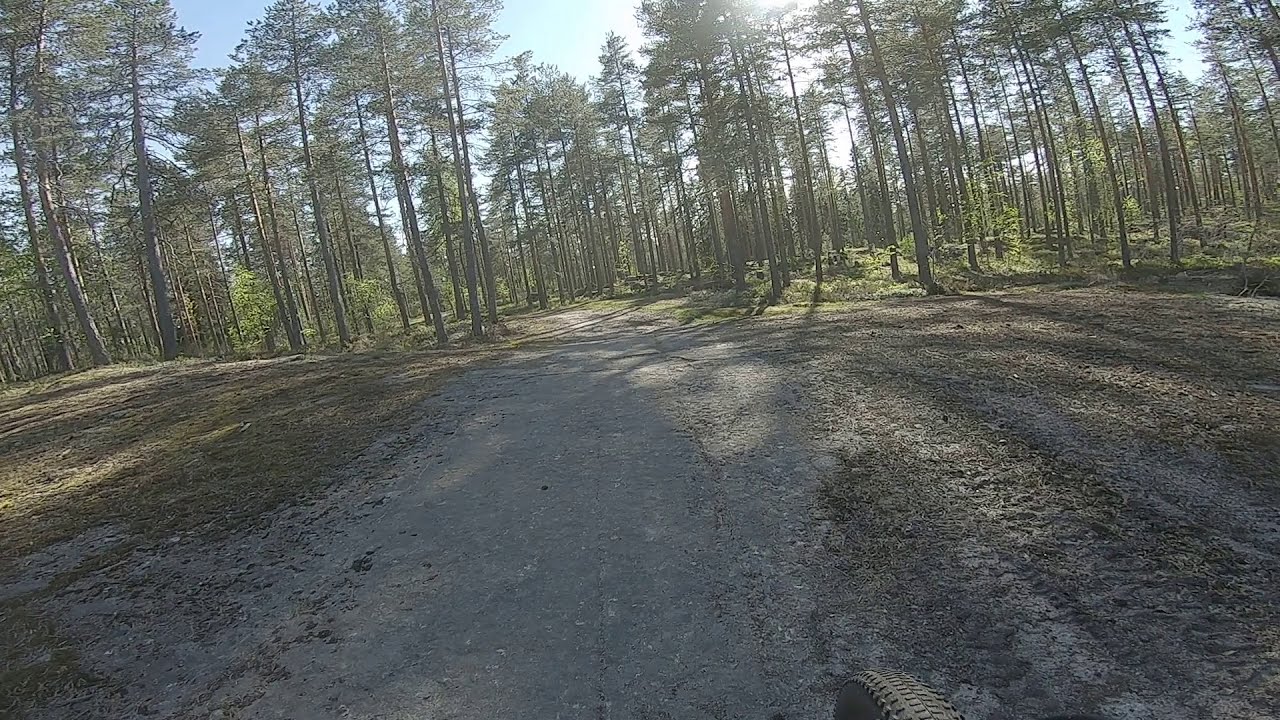This image provides an immersive perspective of a bike ride through a dense, towering forest, captured presumably from a GoPro mounted on the rider's helmet. Starting at the bottom right corner, a faint glimpse of the front wheel suggests the rider's presence on a dirt bike, gliding over a compacted gray dirt trail that cuts through the woodland expanse. The trail meanders from the lower frame, curving into the forest and disappearing among the trees. The ground on either side of the trail is covered in short, muddy brown grass, giving way to a mix of mossy patches. Flanking the trail are countless slender trunks of pine or another type of evergreen tree, consistently shooting straight up with sparse branches until much higher up, where dense green needles cluster, allowing occasional glimpses of the blue sky above. About halfway up the frame, the forest's density increases, creating a canopy that envelops the scene in a serene, verdant embrace.